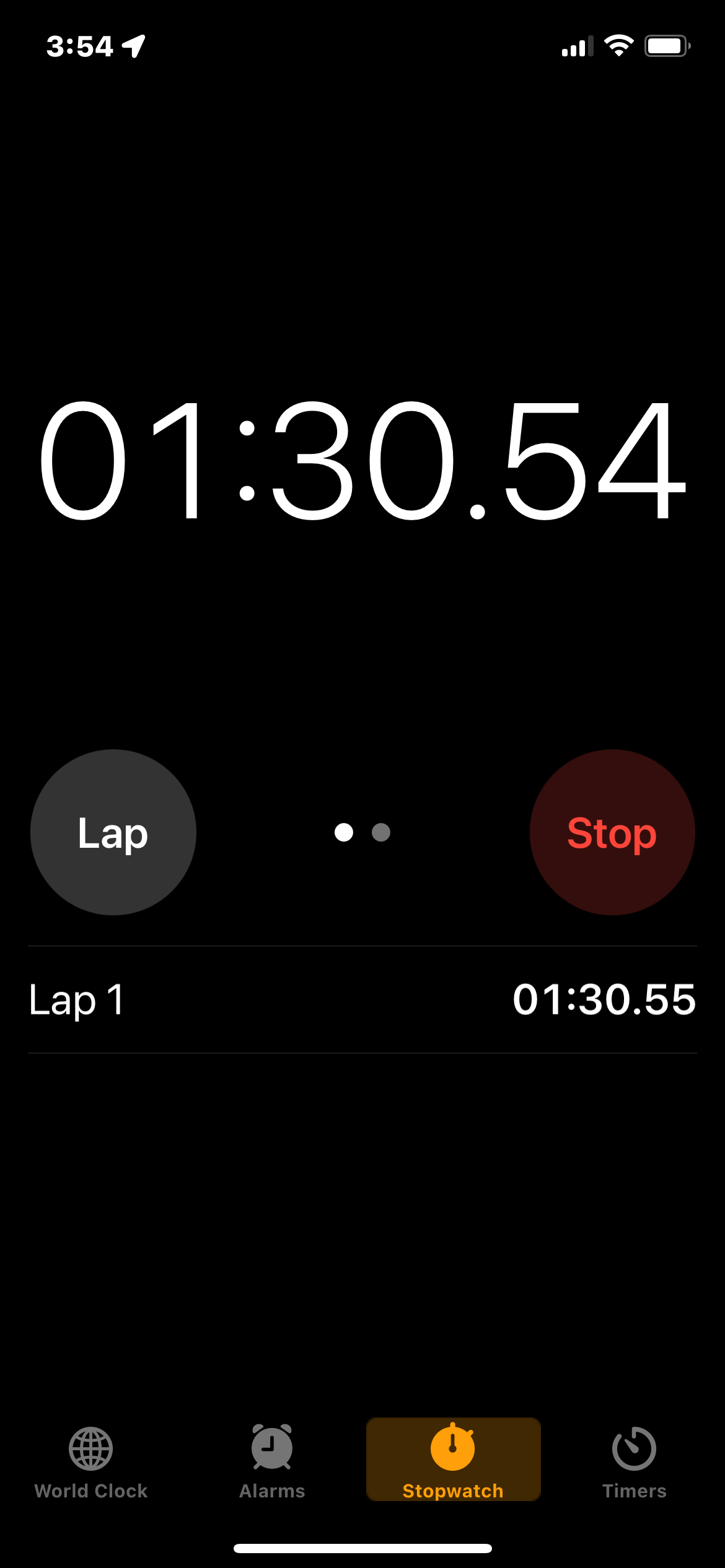This screenshot captures a cell phone's stopwatch interface. The background is black, providing a stark contrast to the white font used throughout. In the upper left corner of the screen, the current time is displayed as 3:54, with a GPS pointer icon to its right. On the upper right, indicators show three bars of cell phone reception, full Wi-Fi signal, and a nearly full battery at approximately 98%.

Beneath these status icons is a large, empty black space. Dominating the center of the screen is the stopwatch readout, prominently shown in large white font as "01:30.54." Below this, smaller text denotes a lap with the label "Lap 1." Further down, the text "Stop at 1.35 seconds" is displayed, likely indicating the time for the most recent lap.